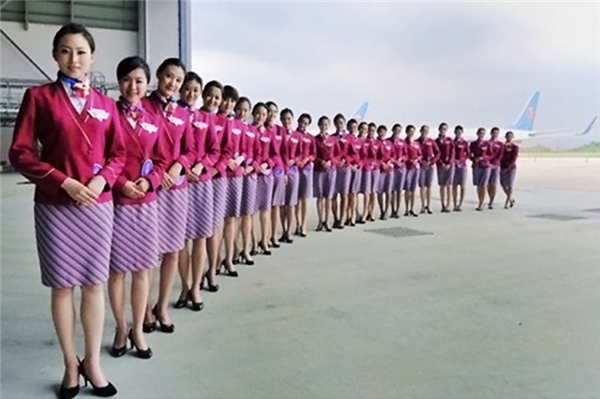In this image, a group of 25 Asian female flight attendants are lined up in a semi-circle formation on a gray tarmac, near the entrance of a hangar with its doors fully open. Dressed uniformly in magenta jackets adorned with white handkerchiefs or neck sashes, they also sport purple skirts featuring diagonal stripes in various shades of lilac. Each attendant is wearing black high-heeled shoes. They stand with their arms slightly overlapping at their midsections, giving a cohesive and professional appearance. In the background, partially visible aircraft, including the tails, wingtips, and rear elevators, can be seen against the backdrop of the airport. The attendants are positioned such that those in the front are more illuminated, while those inside the hangar appear darker due to the lighting difference.